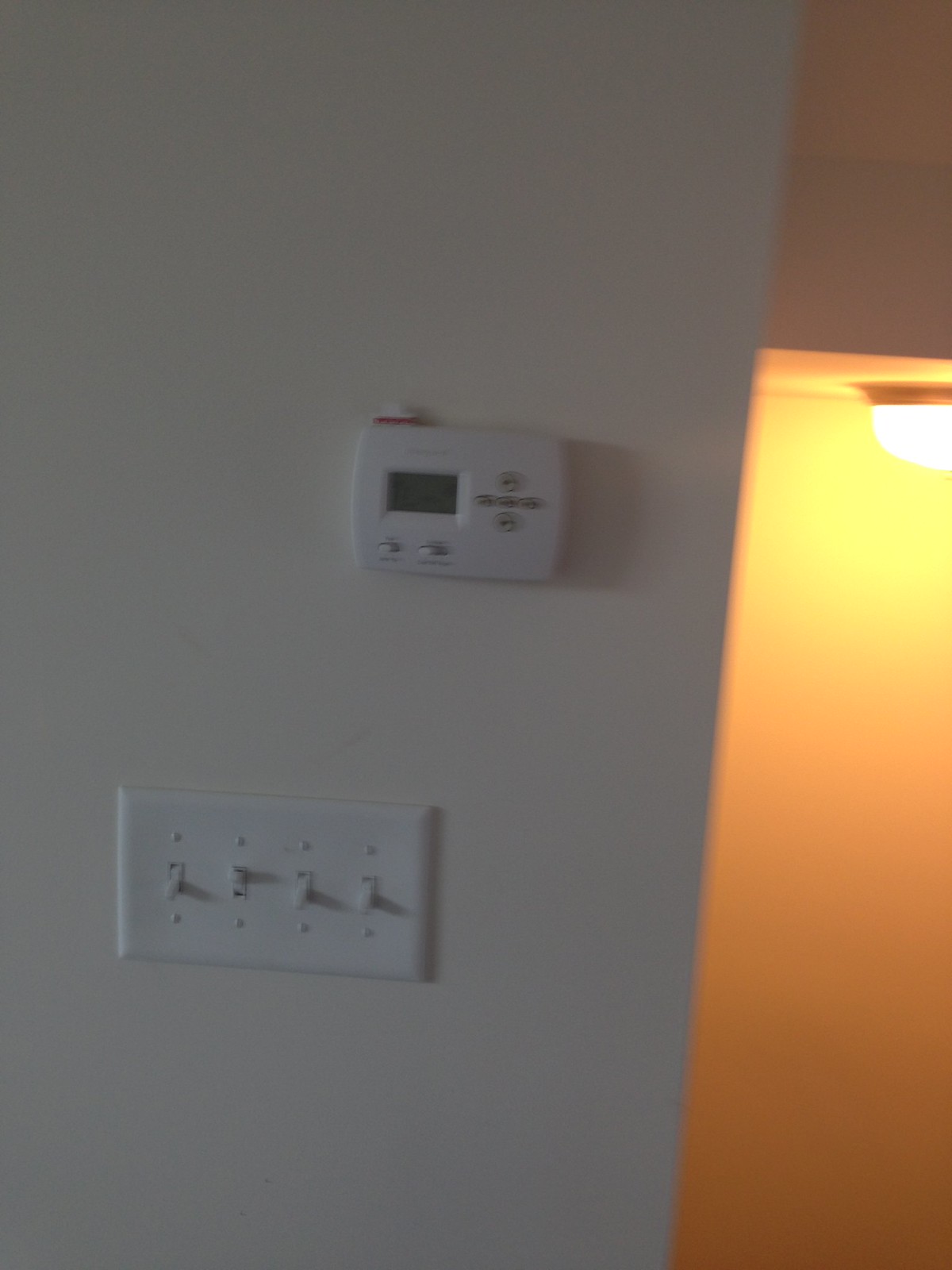This photograph captures the interior of a home, focusing on a section of a white wall adorned with a few notable features. Mounted slightly off-center to the right is a white plastic thermostat, characterized by a small LCD display on its left side. Beneath the display are two tiny switches that can be toggled left or right, and to the right of these switches are four directional buttons labeled with upward, downward, leftward, and rightward arrows. Due to the photo's poor quality, the text on the digital display is unreadable. Below the thermostat, a four-gang light switch plate sits flush against the wall, painted in the same white color for a seamless look. Out of the four switches, all are in the downward 'off' position except for the second switch from the left, which is flipped upward. To the lower right of these wall-mounted elements is a recessed niche illuminated from the top by a silver-base light fixture with a round bulb, adding a subtle glow to the alcove.